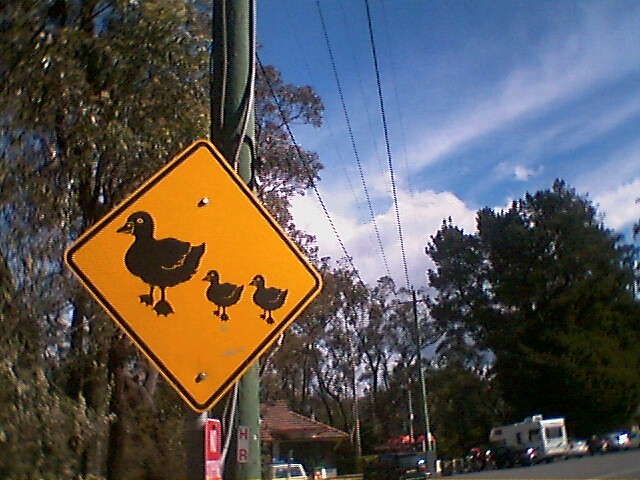The image features a yellow road sign mounted on a green pole, depicting a mother duck followed by two ducklings, indicating a frequent duck crossing area. The environment surrounding the sign includes tall trees, a camper van, multiple parked cars, and a small building that resembles an information center, suggesting the location might be a campground or a residential neighborhood. The asphalt surface of either a parking lot or roadway is visible beneath the sign. The background showcases a blue sky adorned with wispy clouds and intersected by power lines, emphasizing the main focus on the duck crossing sign.